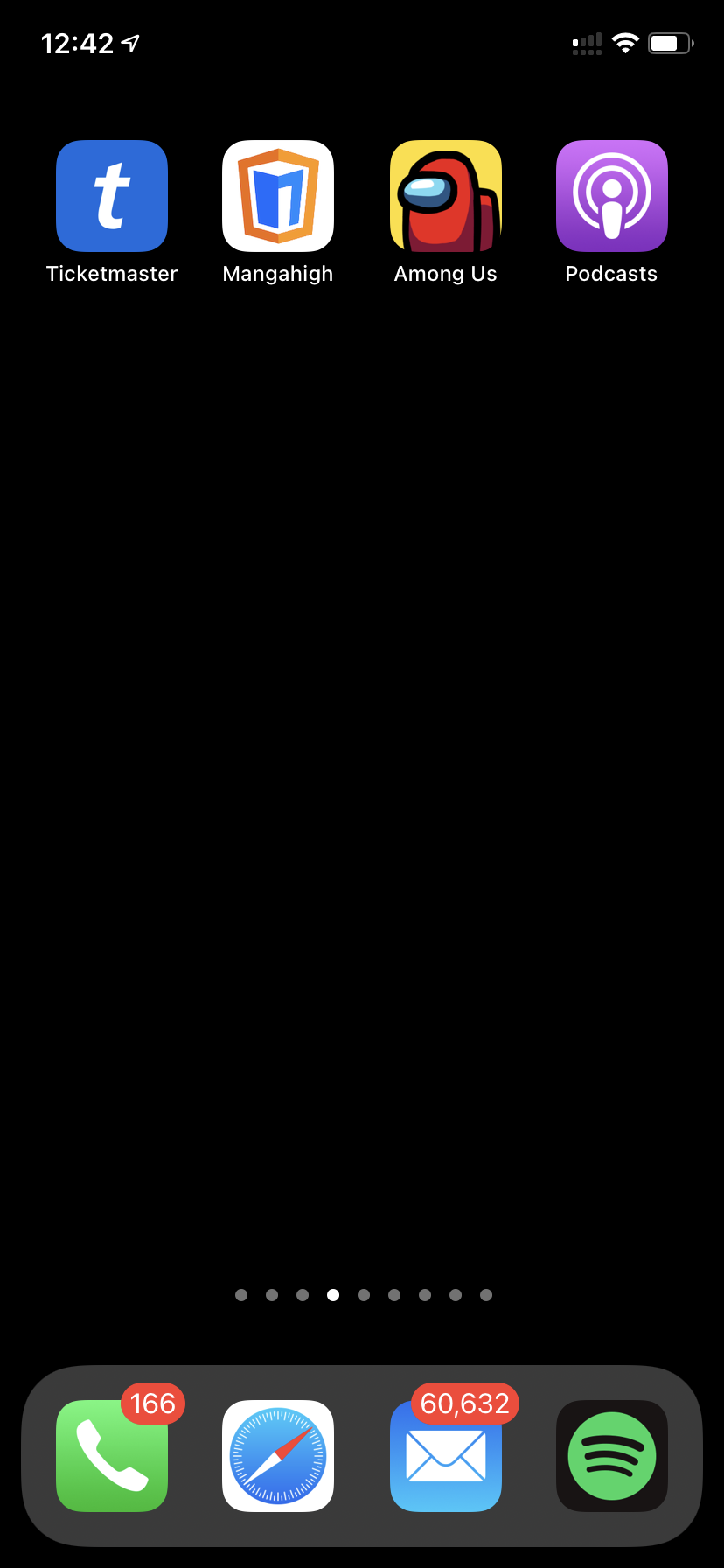The screenshot from a phone display shows the time as 12:42. The signal strength is low with only one bar, but the Wi-Fi icon indicates a strong connection. The battery level is approximately three-quarters full. The background is black, and there are four prominent app icons lined up.

1. The first app on the left is Ticketmaster, represented by a blue box with a lowercase white 't' in the middle.
2. Next to it is Mangahigh, depicted by a white box featuring an orange hexagonal border. Inside the hexagon is a blue geometric shape with a chunk missing on the right side, creating a dip in the middle at the top.
3. The third icon is for an unknown app, presenting a yellow box with two red, semi-circular shapes and a gray oval on the left shape.
4. The fourth app is Among Us, showing a yellow box with two red, semi-circular shapes resembling crewmates from the game.